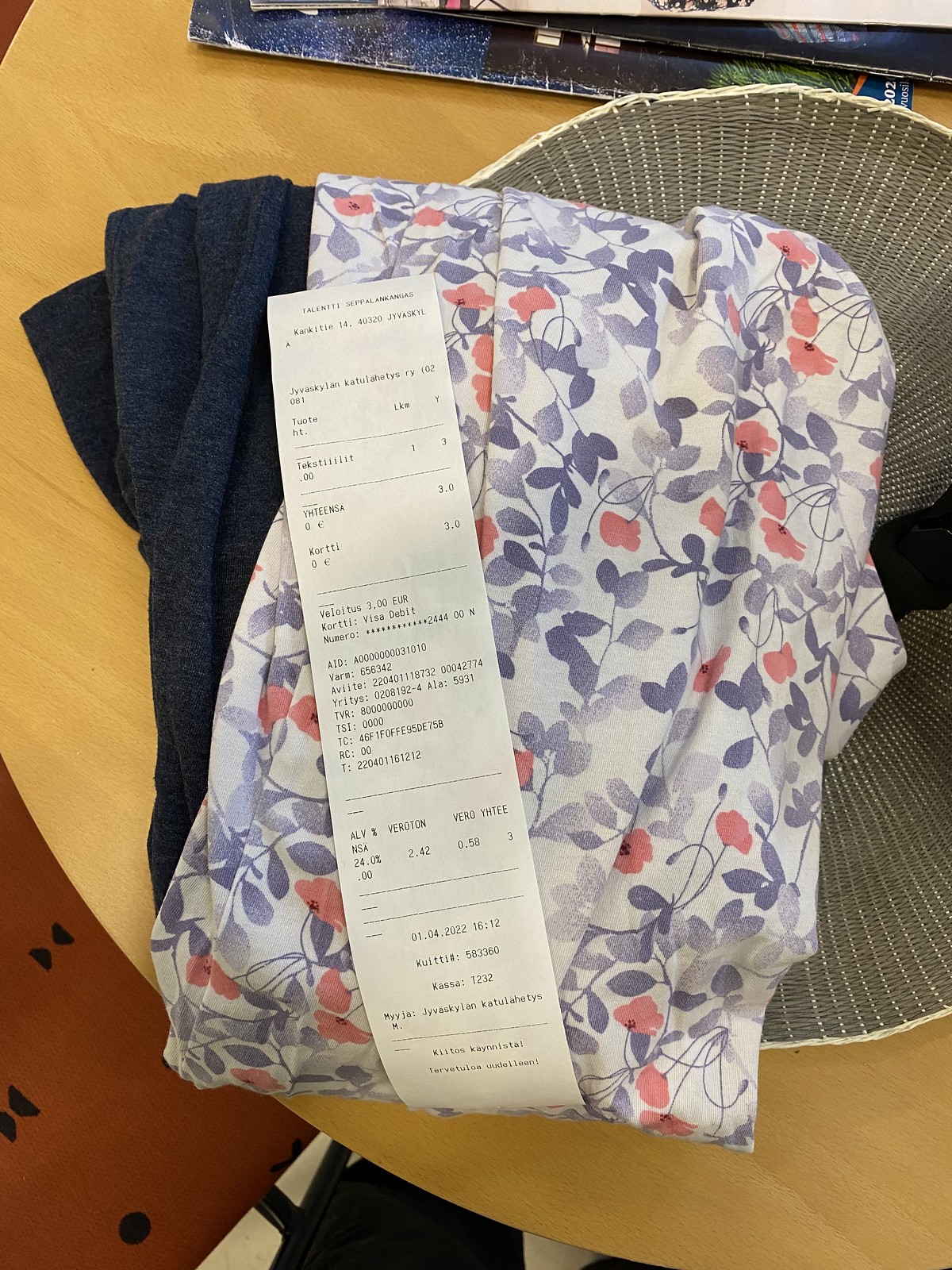This color photograph shows an array of objects carefully arranged on a partially visible round, beige wooden table. Dominating the scene is a large circular white basket filled with neatly folded clothing. The bottom layer of the basket contains a dark gray fabric, possibly a piece of clothing, partially obscured by a white garment adorned with a blue and orange floral design. Draped vertically from the top edge of the fabric to its bottom is a long white receipt with tiny, unreadable black text, except for the discernible word "Reza Debit" and some foreign words like "T-A-L-E-N-T-T-I" and "S-E-B-P-P-A-L-A-N-K-A-N-G-A-S." Just peeking above the top edge of the basket, in the very upper corner of the image, is a blue rectangular object that might be a book or an electronic device such as a laptop. The pile rests on what appears to be a grey place mat with a round white edge. The background includes a red surface beneath the table and a black and white surface towards the lower edge of the image, with a possible back of audio equipment slightly emerging at the top of the shot.